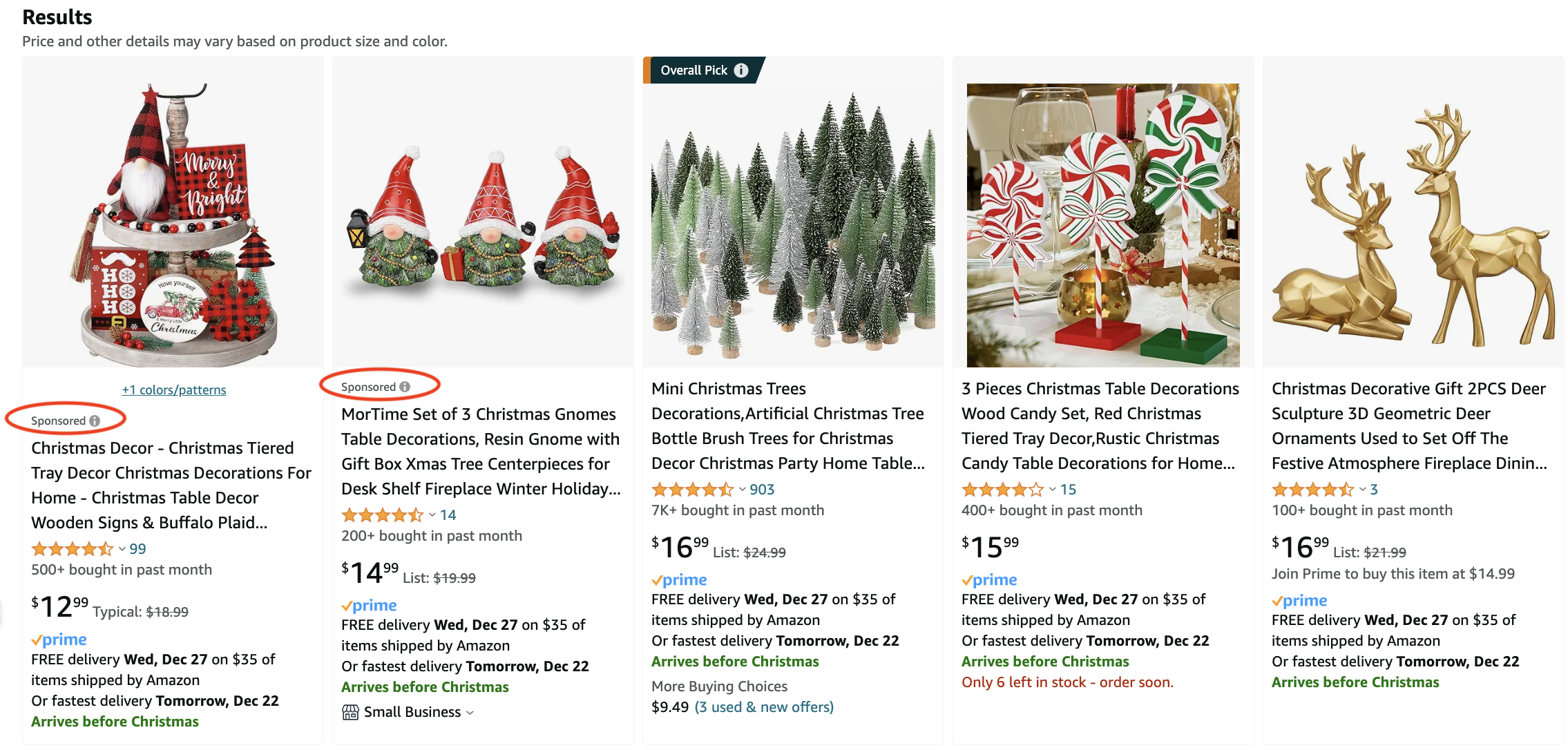The screenshots depict various Christmas decorations available on Amazon. The search results include a variety of festive items, starting with a sponsored ad for a charming miniature Christmas house, resembling a gnome house, priced at approximately $13. Another sponsored ad showcases a trio of whimsical Christmas gnome table decorations available for around $15.

Following that, there is an offer for artificial mini Christmas trees, suitable for decoration purposes, listed at $17. In another screenshot, a three-piece set of wooden candy cane table decorations is priced at $16, adding a playful touch to the holiday decor.

Additionally, there are intricately designed reindeer sculptures, marketed as 3D deer decor, also priced at $17. The listings all indicate free delivery by December 27th, with a specific note mentioning delivery by tomorrow, December 22nd, suggesting the user was browsing these options on December 21st, in the lead-up to Christmas, presumably aiming to add more festive decorations to their home.